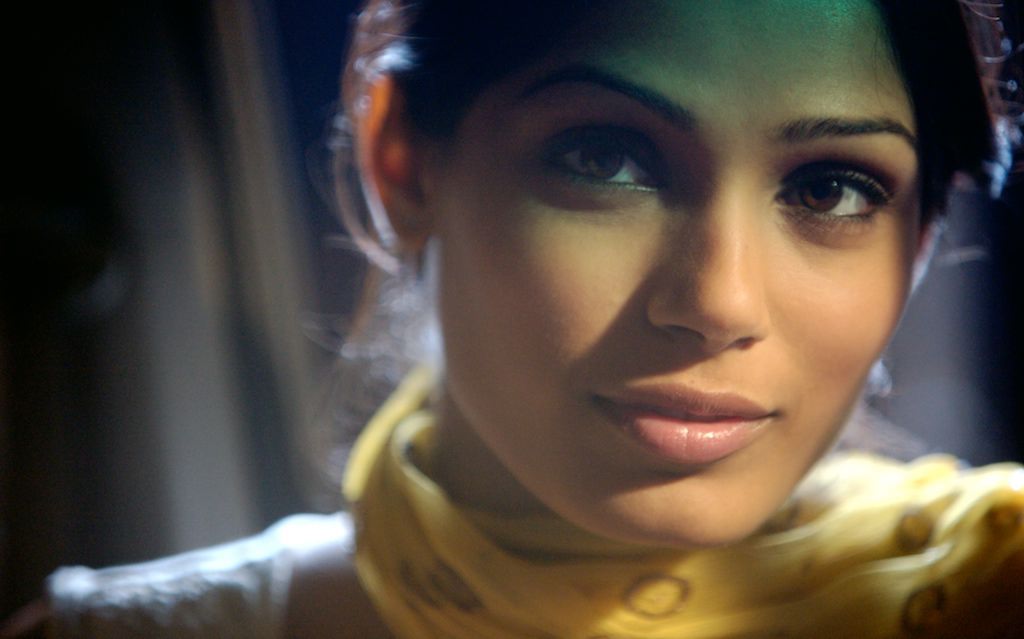This is a close-up, horizontal rectangular photograph of a very attractive young woman, likely in her mid to late 20s, with a brown skin tone and striking features. The image is cut off at her forehead, emphasizing her expressive brown eyes that are framed by penciled eyebrows, and she is wearing lipstick along with other makeup to highlight her natural beauty. She has dark hair, which is visible only in one corner, suggesting it is pulled back. She is wearing a soft gold or yellow scarf around her neck that drapes over one shoulder. The lighting in the photograph casts a shadow from her nose, indicating overhead lighting that highlights the top of her shoulders while leaving areas below in shadow, suggesting her attire might be a light-colored blouse or jacket, though the exact details are obscured by the darkness and shadow. The background is very dark with indistinct line patterns resembling a curtain, focusing attention solely on the woman, who is smiling subtly, giving a somewhat seductive or smirking expression.